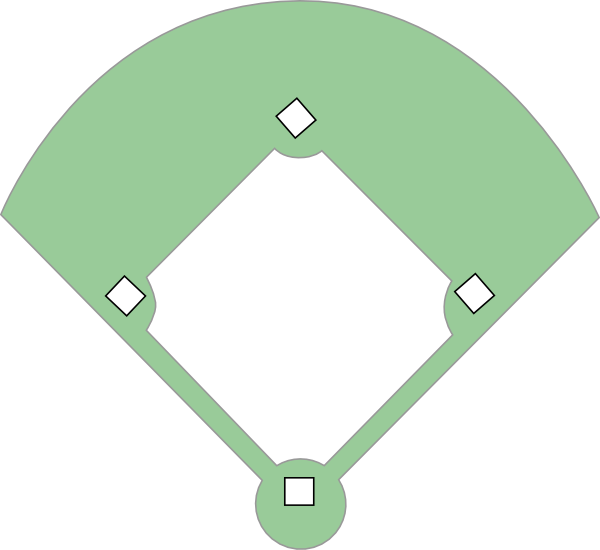The image depicts a simplified sketch of a baseball diamond on a completely white background. The infield section is entirely white, featuring home plate, first base, second base, and third base as white squares outlined in black. Notably, first base, second base, and third base are rotated 45 degrees, presenting as diamond shapes from our perspective. There is no visible pitcher's mound. The outfield and base paths are colored in a light green or slightly bluish-green hue, which stands out against the stark white infield. The green area forms a semi-circular shape around the infield, curving from right field to left field and peaking at center field, creating an overall image resembling the layout of a baseball field. However, this is clearly a simple, illustrative sketch rather than a detailed, realistic representation. There are no players or additional field details depicted in the image.